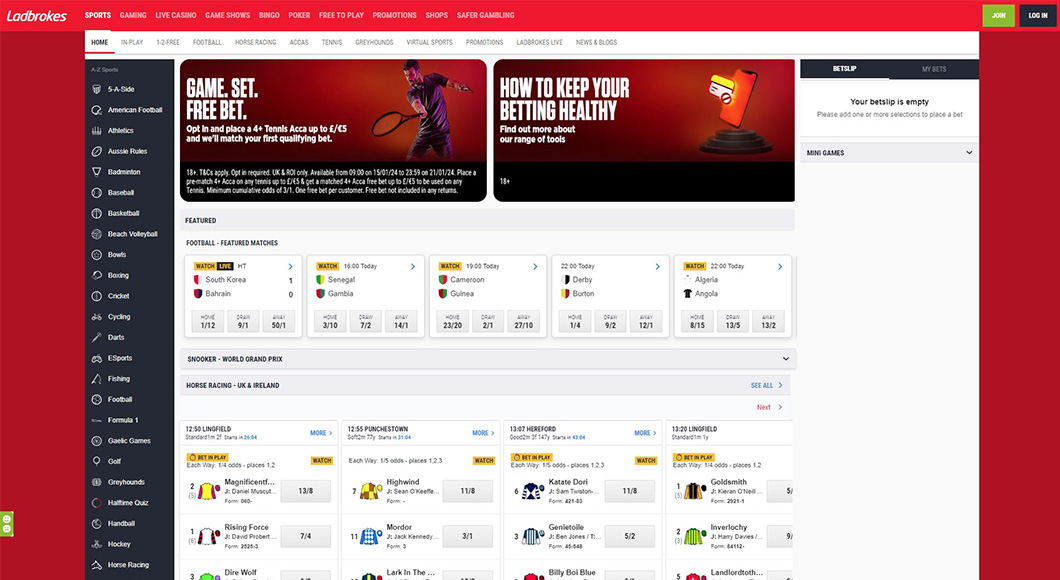The image showcases a website with a vibrant red background that transitions to a brighter red at the top. Prominently displayed at the upper section is the word "LADBROKES" in bold, white capital letters. Below this header is a navigation bar with various categories listed: the word "Sports" stands out in bold white text, while the other categories—Gaming, Live Casino, Game Shows, Bingo, Poker, Free-to-Play, Promotions, Shops, and Safer Gambling—are in regular white font.

Beneath this, a white banner presents additional menu options, though some are blurred. The visible options include Home, In-Play, 1-2-3, Football, Horse Racing, ACCAS, Tennis, Greyhounds, Virtual Sports, Promotions, Ladbrokes Live, and News & Blogs. Towards the left of the banner is a menu icon, beside a black banner housing two images. One image states "Game Set, Free Bet," focusing on promoting responsible betting practices. The other image provides statistics and matchup details for various ongoing games and events.